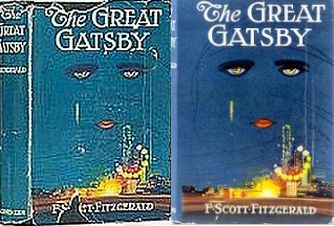The image consists of two covers of the classic book, *The Great Gatsby* by F. Scott Fitzgerald, displayed side by side. Both covers are predominantly blue and feature the same distinctive artwork, which includes two melancholy eyes, red lips, and what appears to be a tear. Below these facial elements, there is a cityscape with yellow lights or explosions resembling a carnival scene. The title "The Great Gatsby" is prominently displayed at the top of both covers, while the author's name, "F. Scott Fitzgerald," appears at the bottom, albeit with damage in different degrees on each cover.

The book on the left shows significant signs of wear, with heavy damage to the cover including rips and tears that obscure parts of the author’s name, leaving only the last letters "-gerald." The cover also exhibits wrinkles and overall looks older. It also slightly reveals the spine of the book, which also displays the title "Great Gatsby." The book on the right, though somewhat blurry, is in relatively better condition with less damage, presenting a clearer view of the author’s full name and the cover art intact. Both covers share the same iconic imagery and text, but the left one’s condition makes it appear more worn and aged.